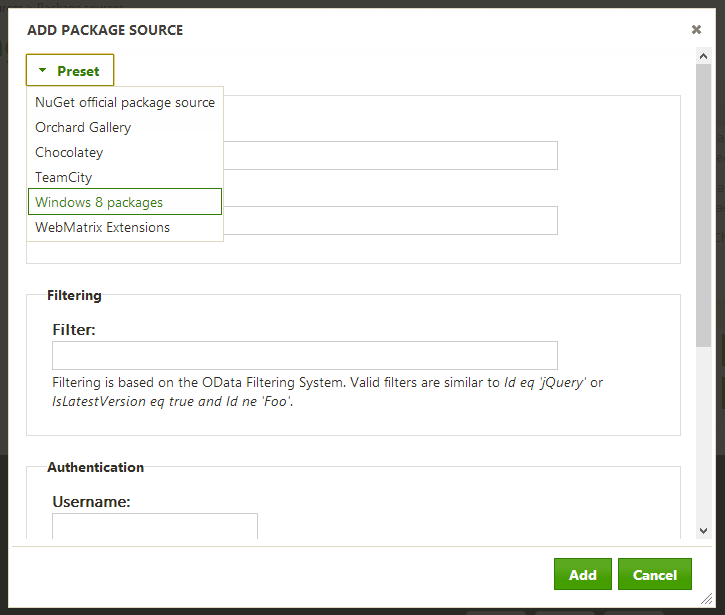**Detailed Description of the Interface Window**

The interface window features a thick black border and is square in shape. Located at the top left, the title "Add Package Source" is displayed prominently in bold, black capital letters. Directly below the title is a dropdown menu, bordered in a yellowish-green hue. The dropdown menu includes a bold, green dropdown arrowhead icon with the label "Preset," also in bold green lettering.

The dropdown menu presents several options: "NuGet Official Package Source," "Orchid Gallery," "Chocolatey," "Team City," and "Windows 8 Packages." The currently selected option, "Team City," is highlighted in green text and outlined with a green border for emphasis. Below this, the menu continues with "Web Matrix Extensions," rendered in standard black text without a border.

Behind the dropdown menu, two editable fields are visible but partially obscured by the dropdown window. Below the fields, another section labeled "Filtering" appears in bold black letters. This section includes a "Filter:" label followed by an editable text area. In gray lettering, an explanatory note reads: "Filtering is based on the ODATA filtering system. Valid filters are similar to 'ID EQ 'JQuery'' or 'IsLatestVersion EQ true' and 'ID NE 'FOO'."

Adjacent to this section, another area is labeled "Authentication" or sometimes "Authentication" in bold lettering. The accompanying field for "Username:" is also marked in bold, located towards the left, with the input area outlined by a light gray border.